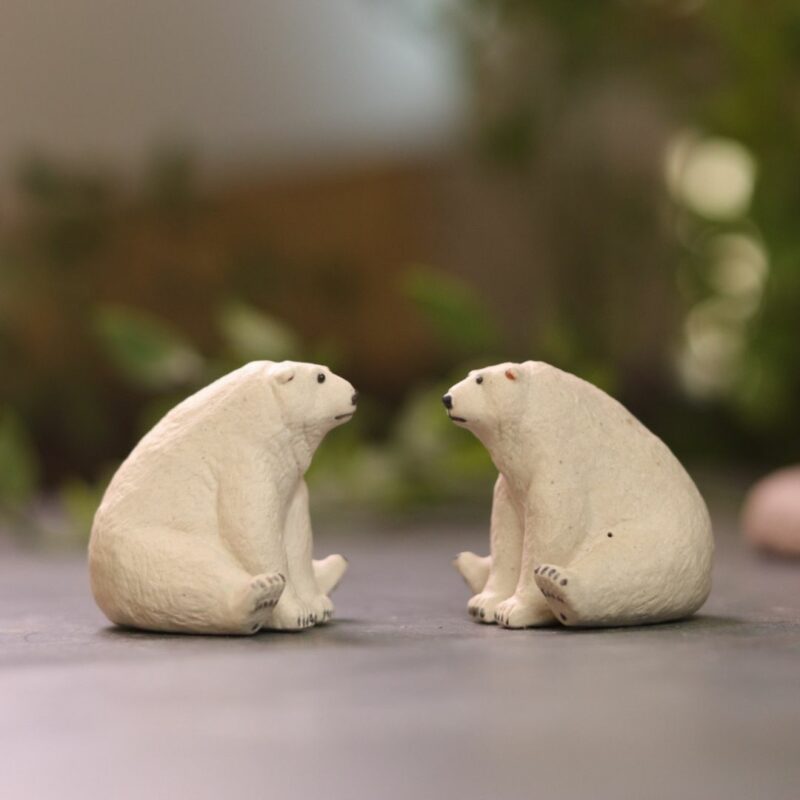The image is a large, detailed square showing two small figurines of polar bears in the center, facing each other. Each bear is sitting on its haunches on a gray surface, with their front paws positioned between their splayed back paws. Both figurines are predominantly white with small black details, including tiny black dots for eyes and noses, a thin black line for a mouth, little black lines indicating claws, and some black shading on the pads of their feet. The polar bears have distinct facial features: one has a higher, rounder snout than the other. They also have slightly red-tinted inner ears. The figurines appear to be made of ceramic or possibly painted stone. The backdrop is blurred, revealing vague hints of greenery and white, likely foliage and light reflections, set against the suggested shape of a wall. This subtly blurred background ensures that the main focus remains on the intricate details of the polar bear figurines.